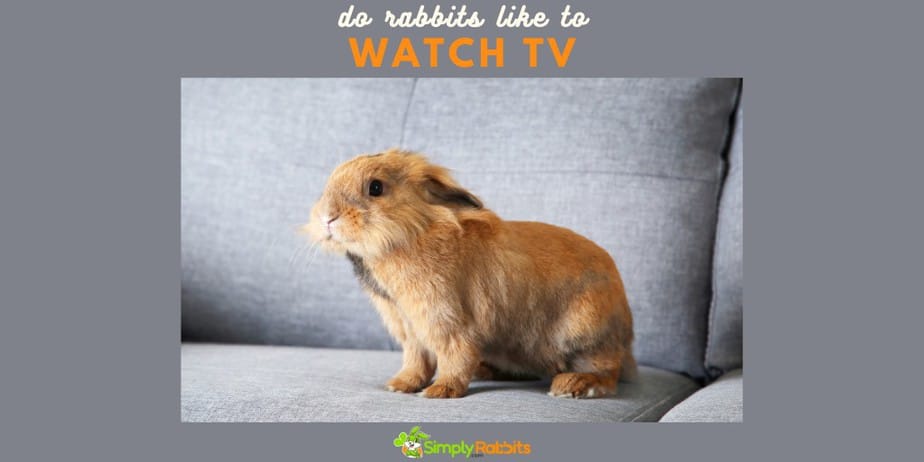The image consists of a dark gray background enveloping the top, left, right, and bottom edges. At the top, elegantly written in cursive white letters, appears the question: "Do rabbits like to". Just below this, in bold orange capital letters, it reads: "WATCH TV?". The bottom portion of the image features a cartoon illustration of a rabbit with distinctive features. The rabbit has green ears and appears to be wearing an orange shirt. Below the rabbit illustration, there is text in green handwriting-style letters and bold orange letters that says: "Rabbits". 

Above this text, there is a zoomed-in area focusing on a section of a sofa, revealing just the seat and backrest, shaded in gray. Seated on the sofa, prominently positioned, is the rabbit character. The rabbit has its ears laid back against its head and is looking to the left side of the image. The rabbit's fur appears to be a blend of brownish-red color, it has a pink nose, and its tail is not visible in the illustration.